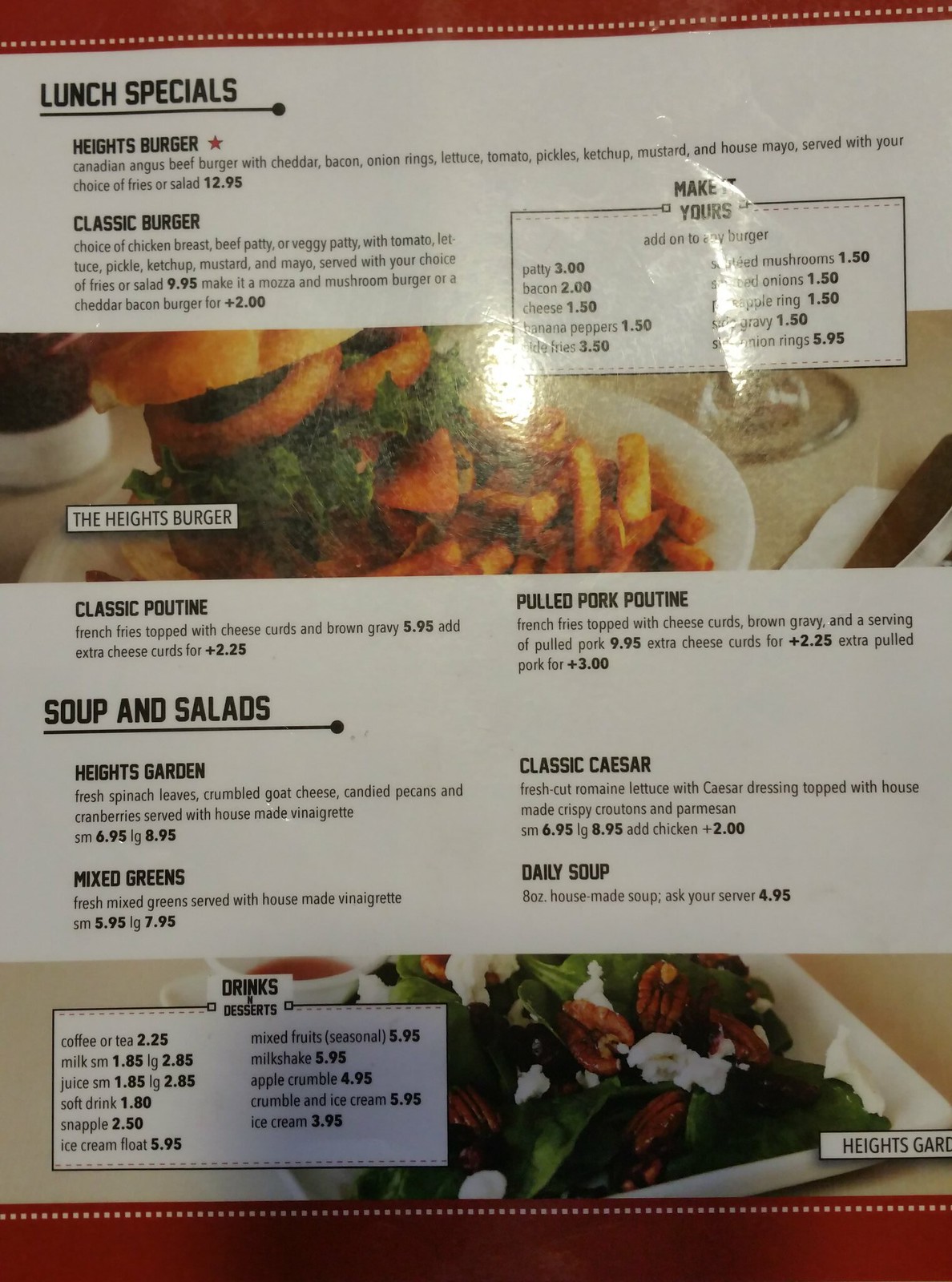This photograph showcases a laminated paper menu, which features a glossy surface reflecting light in two sections located in the upper right corner. The menu itself is designed with white paper and accented by thin dark red borders at the top and bottom. These borders are adorned with small white dots, arranged in a stitch-like pattern along the inner edge.

The menu is divided into two primary sections. The upper section, titled "Lunch Specials," lists several items in bold font with detailed descriptions in smaller font beneath each item. The lower section, "Soups and Salads," follows the same formatting style.

Two images are prominently displayed on the menu. The first image, located about two-thirds up the menu, is presented as a banner stretching across the width. It features the "Heights Burger," a tall burger topped with onion rings, lettuce, and tomatoes, accompanied by a pile of French fries on a white plate. 

The second image, positioned in the lower section, depicts a square white plate filled with a spinach salad garnished with pecans and crumbled white cheese, likely feta. This dish is labeled "Heights Guard," likely intended to be "Heights Garden Salad," though the name is partially cut off by the edge of the photograph.